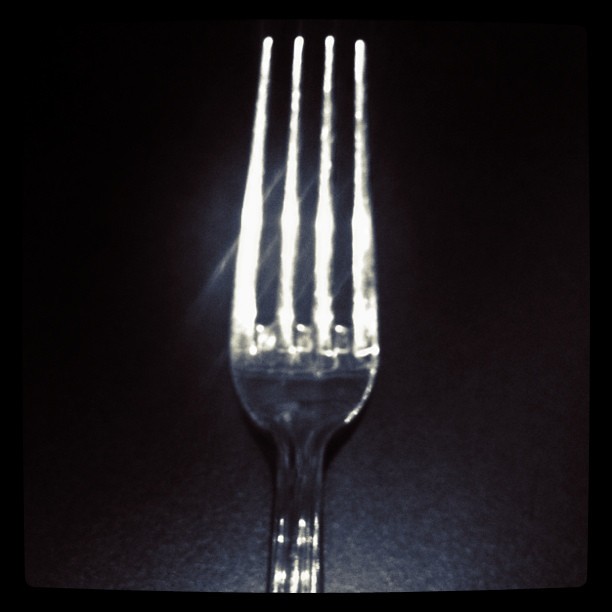This black and white photograph captures an extreme close-up of a stainless steel fork set against a pitch-black background. The fork, featuring four reflective tines, is centrally aligned and appears to extend vertically down the middle of the image, with an inch of its handle visible before it disappears beyond the bottom edge of the frame. The prongs gleam under a bright light source, creating stark white highlights that fade into gray shadows along the rest of the fork. The varying shades lend a textured, almost gradient effect to the steel, emphasizing the contrast between light and shadow. Despite the uniform darkness of the background, the light creates subtle variations and reflective lines around the fork, enhancing its distinct metallic sheen. The handle and the lower part of the fork exhibit darker tones, adding depth to the composition while maintaining the fork's silvery essence.